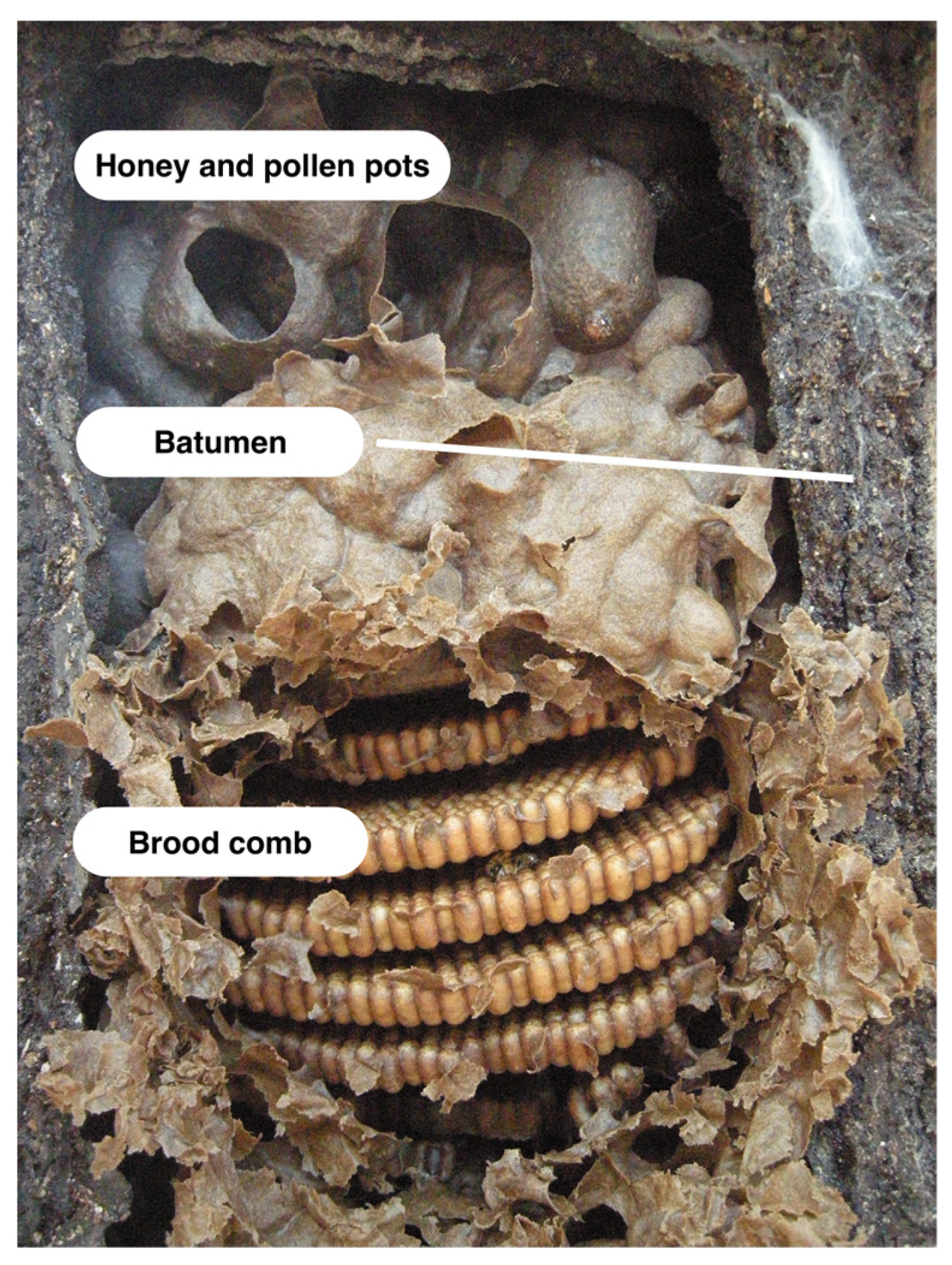This detailed image reveals the dissection of a beehive nestled within a tree hollow, exposing its intricate internal structure. The beehive is encased in a grayish outer layer labeled "batumen," presumably serving as the protective exterior. At the top, the label "honey and pollen pots" identifies round, bulbous containers, some of which appear broken open, with honey visibly leaking out. Below these pots hang brown sacks that blend into the surrounding structure. Toward the lower section of the hive, a series of horizontal disks resembling wheels or rows of corn—identified as "brood comb"—are where bee larvae develop. This image, while intriguing, also evokes a sense of the unusual and alien, presenting the beehive's complex and somewhat eerie appearance.